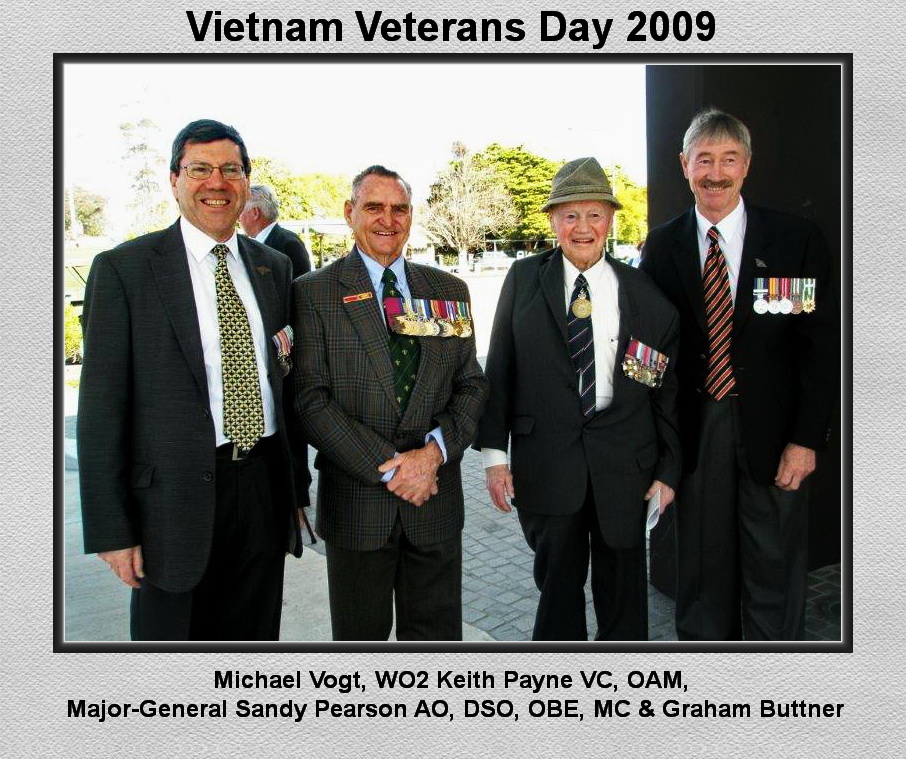The image depicts a photograph bordered in gray, showcasing four elderly Caucasian men standing side by side and facing the camera at what appears to be a cemetery. The photograph is captioned at the top with black text that reads "Vietnam Veterans Day 2009," and at the bottom with the names and titles "Michael Vogt, W-O-2, Keith Payne, V-C, O-A-M, Major General Sandy Pearson, A-O, D-S-O, O-B-E, M-C, and Graham Butner." All four men are dressed in formal suits with ties and adorned with an array of military honors on their lapels. 

The man on the far left is of medium height, wears glasses, and is dressed in a dark gray suit paired with a white shirt and a yellow and black tie. To his right is a shorter, slightly older man in a deep gray pinstripe suit and green tie, displaying a row of medals on the left side of his chest. The third man from the left dons a dark green hat and is attired in a dark suit with a black pinstripe tie, also heavily decorated with medals. The man on the far right is the tallest, with dark gray hair and a prominent mustache, sporting a dark suit, a red and black pinstripe tie, and medals on his right. In the backdrop is a gray pavestone, a bright white sky, some trees, and a fifth man standing slightly away from the group, facing away from the camera.